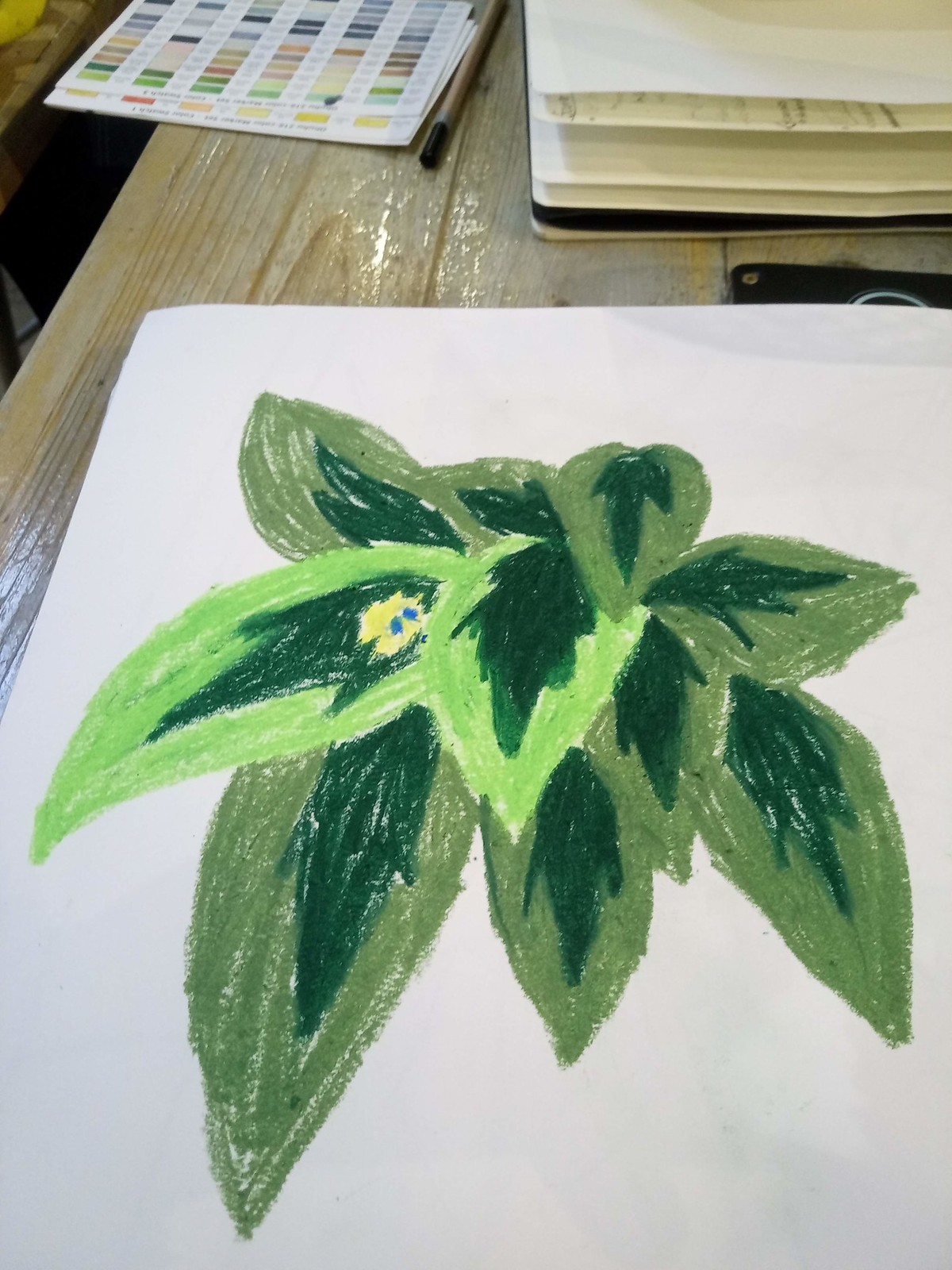This photograph captures a meticulously crafted drawing on a large white sheet of paper. The artwork, likely created using crayons, colored pencils, or possibly pastels, features an intricate arrangement of oversized, teardrop-shaped leaves with pointed tips. The leaves exhibit a vivid gradation of colors, ranging from dark green to lighter green, with a prominent dark green core in the center. The coloring is rich and densely applied. In the background, there is a glimpse of a sketchbook or ledger, bound in white paper, partially visible. To the left of the drawing, a color palette is discernible, hinting at the artist's process. The entire scene is set against a light, almost gray wooden desk or countertop, adding a natural and subtle contrast to the vivid artwork.